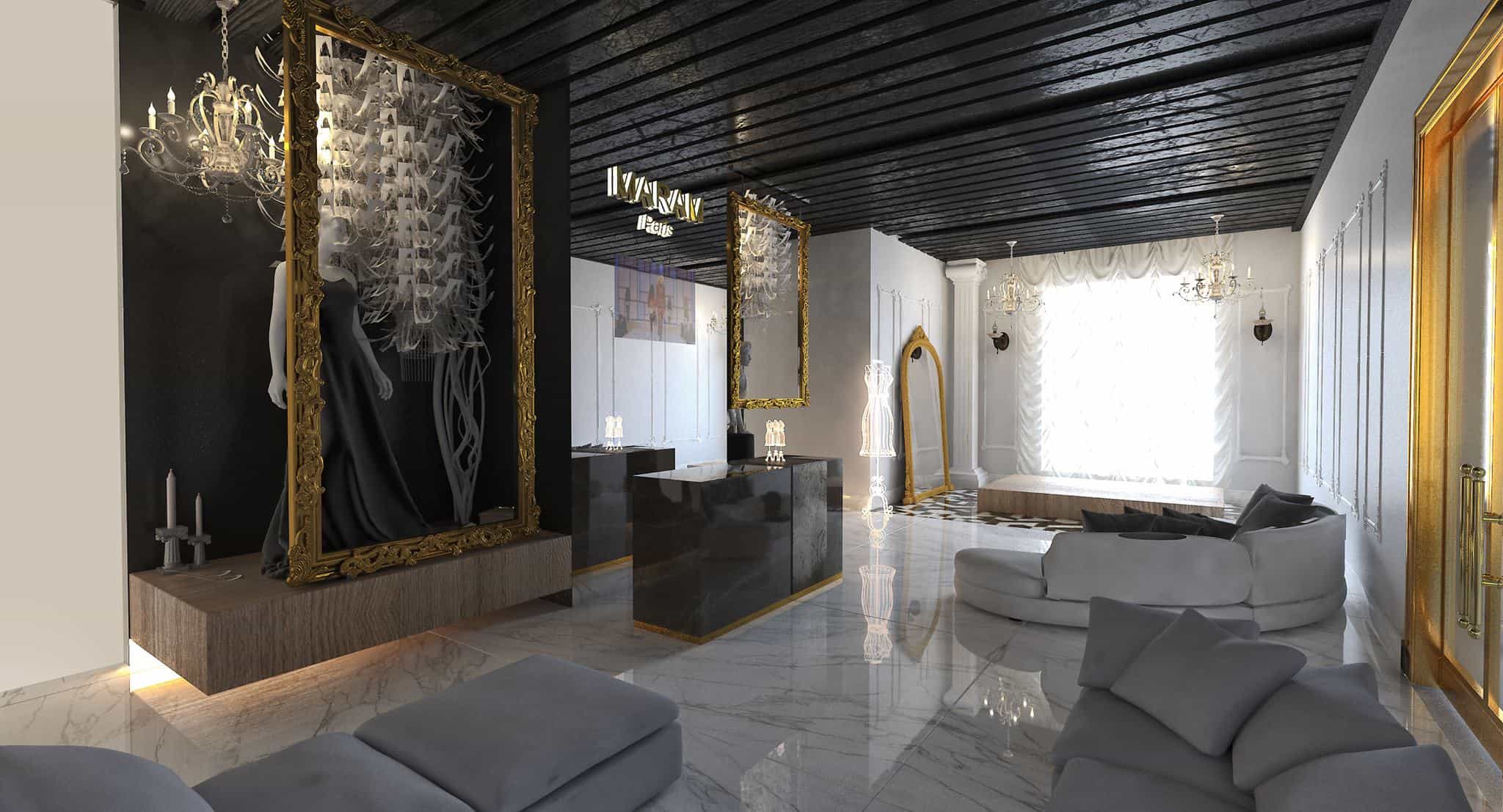The image depicts a strikingly elegant and modern waiting area, potentially a spa lobby or an elite retail store. The room features a polished white marble floor accented with faint black streaks, enhancing its luxurious feel. Dominating the space are plush, gray, and cream-colored couches, including a semi-circular white couch with gray pillows, all meticulously fluffed for comfort and style.

Central to the room is a gray marble welcome desk that mirrors the sophisticated dark, wooden plank ceiling above. The ceiling contrasts beautifully with the room's white walls and the overall bright ambiance. Various reflective surfaces add depth, such as a large gold-framed mirror or artwork, which, intriguingly, appears to display a mannequin in a formal gown.

Behind the mannequin, a hanging lamp and two vertical fixtures add subtle details, while other walls boast more gold-framed mirrors and a prominent column. The entrance possibly features lengthy door handles, hinting at a grand entry. Complementary chandeliers throughout the room shine over the sleek, modern decor, further emphasizing the high-end sophistication of the setting. The welcoming atmosphere is softened with translucent white drapes covering large square windows, completing this exquisitely designed space.